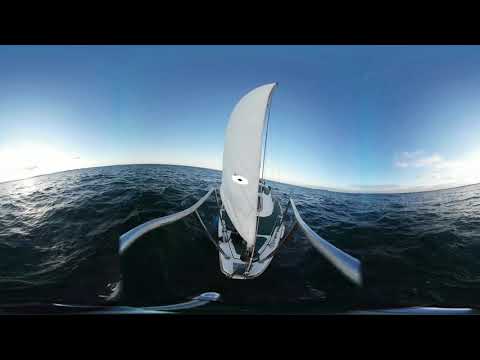The image depicts a slightly distorted photograph of a white sailing yacht, taken at sea. The distortion, likely caused by a fisheye lens, gives the ocean a wavy appearance, with the horizon curving up at the center and then dipping toward the sides. The sapphire blue water is choppy but serene, reflecting the deep hue of the open ocean under a light blue sky that transitions to a darker blue higher up. The yacht is centrally positioned in the image, and is leaning slightly to the left. It features a large, prominent white sail in the middle, extending upwards from a metallic pole. On both sides of the yacht, there are silvery metallic rails stretching outward from the boat towards the viewer, adding a dynamic perspective. The main deck appears bluish-green, possibly carpeted with astroturf. The horizon showcases some white clouds and a sun near the upper left of the image, casting a gentle illumination. The entire scene is framed by a thin black border at the top and bottom, emphasizing the entirety of this oceanic vista.